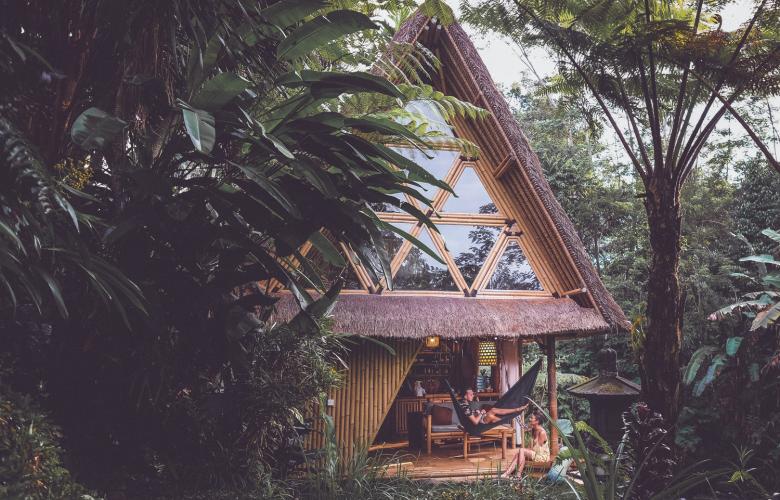The image captures a luxurious A-frame treehouse cabin nestled in the dense, green foliage of a jungle or rainforest. The structure is made primarily of bamboo with a thatched roof that extends over a porch area, adding to its rustic appeal. The roof has large triangular windows divided by wooden beams, creating multiple smaller triangles. The scene is vibrant with lush greenery, including palm trees, banana leaves, and other tropical vegetation that almost obscure the surroundings.

The front of the treehouse features a patio space where a couple is seen relaxing. The man is lounging in a black hammock, which is tied between a column and an exterior wall of the cabin, while a woman in a yellow dress sits on the ground, leaning against a post. Their conversation adds life to the tranquil setting. Behind them, the porch area reveals a cozy environment with a sofa and what appears to be a bar area, illuminated by a hanging lampshade. The ambiance is serene and slightly dim due to the thick canopy of trees above, creating a peaceful retreat within the vibrant jungle.